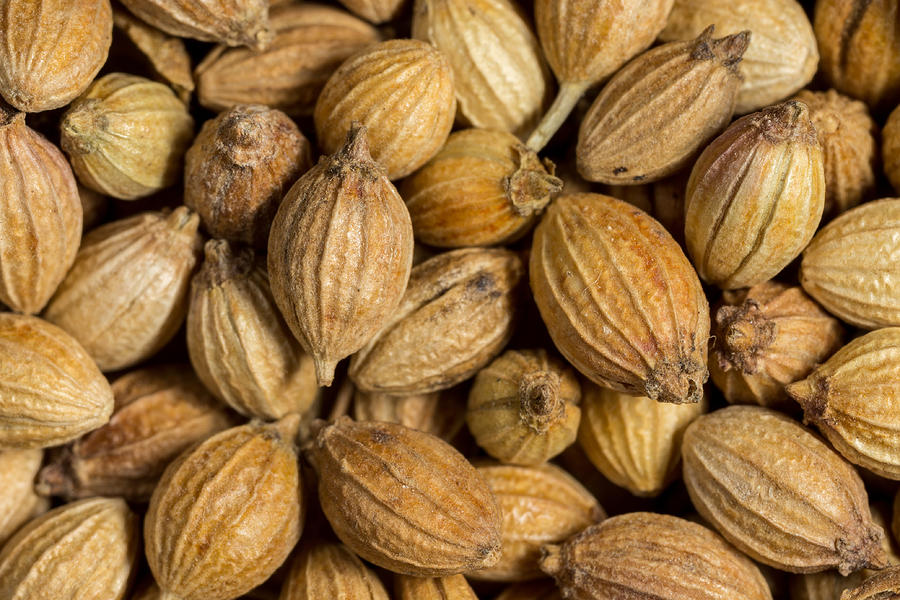This close-up image captures a pile of oval-shaped seeds or nuts, which resemble peanuts or perhaps small pumpkin seeds. Each seed displays vertical ridges or veins running from top to bottom, giving them a textured appearance. They exhibit a light brown to tan coloration, with some seeds slightly darker or lighter, suggesting variability in ripeness. Notably, the seeds feature small protrusions at both ends, resembling stems or potential sprouting points, though none are open. The dry, hard exterior hints at an outer shell that might need to be cracked to access the inside. Positioned haphazardly, some seeds lay flat while others stand upright, filling the entire frame and highlighting the intricate details of their uniform yet varied form.